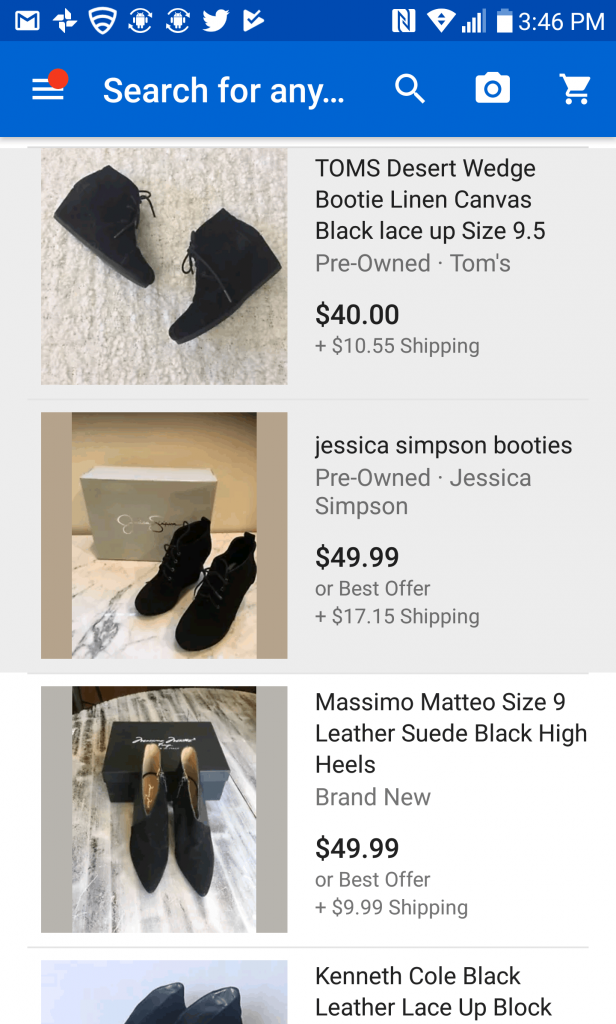The image depicts a screenshot from a cell phone search results page for black boots or black shoes. The top section of the screen features a royal blue background with a search bar containing the beginning of the phrase "Search for any..." along with a small red dot. To the right of the search bar, there are icons for a magnifying glass, a camera, and a shopping cart.

Here are the details of the search results displayed below the search bar:

1. **Tom's Desert Wedge Booty Linen Canvas Black Lace Up Size 9.5**:
     - Condition: Pre-owned
     - Price: $40
     - Shipping: $10.55
     - Seller: Tom's

2. **Jessica Simpson Booties**:
     - Condition: Pre-owned
     - Price: $49.99 or Best Offer
     - Shipping: $17.15
     - Seller: Jessica Simpson

3. **Massimo Mateo Size 9 Leather Suede Black High Heels**:
     - Condition: Brand New
     - Price: $49.99 or Best Offer
     - Shipping: $9.99
     - Seller: Massimo Mateo

4. **Kenneth Cole Black Leather Lace Up**:
     - Text is cut off halfway through the description.

The image clearly captures the structured layout of the search results, providing detailed information about each listing, including price, condition, and shipping costs.